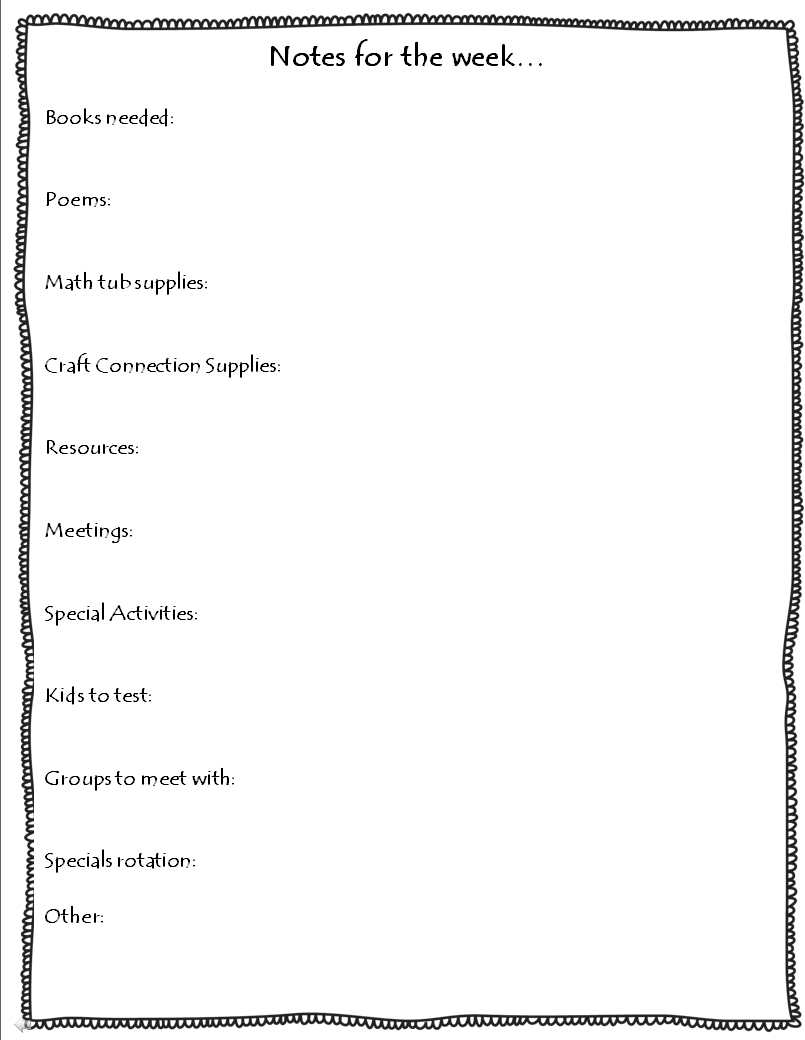This image features a white background with a black border framing the content. At the top of the image, the title "Notes for the Week..." is prominently displayed. Below this title, there is a structured list of categories, each header followed by two dots indicating a space for additional notes. The categories are arranged in vertical order, each item aligned to the left side of the image.

1. "Books Needed.."
2. "Poems.."
3. "Math Tub Supplies.."
4. "Craft Connection Supplies.."
5. "Resources.."
6. "Meetings.."
7. "Special Activities.."
8. "Kids to Test.."
9. "Groups to Meet With.."
10. "Special Rotation.."
11. "Other.."

The text is rendered in a clear, black font which contrasts sharply against the white background, ensuring readability. Each category has ample space next to it for notes or specific items to be listed, which would typically be filled in as required for planning and organization purposes.